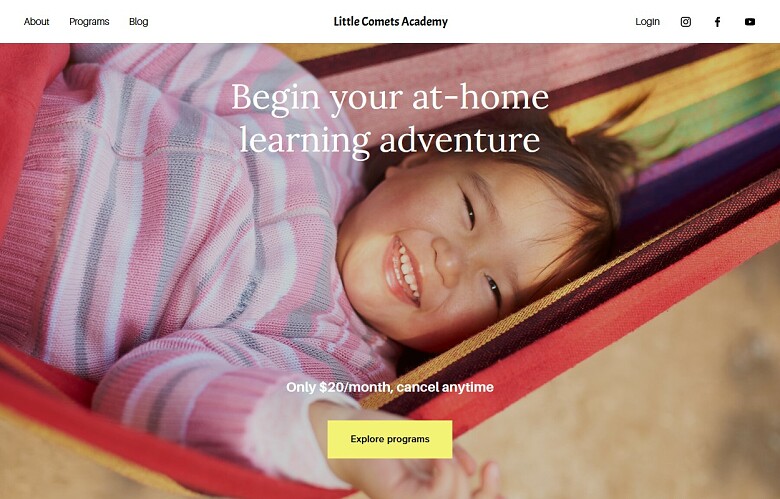The image is a screen capture taken from a desktop computer, showcasing a vibrant web page from Little Comets Academy. At the top-middle portion of the screen, the web page title "Little Comets Academy" is prominently displayed in black text. The focal point of the web page is a colorful photograph featuring a young girl lounging on a lively, multicolored hammock. The hammock boasts stripes in an array of colors, including yellow, green, purple, blue, brown, orange, and lavender.

The little girl, seen from head to waist, has short brown hair and is wearing a cozy striped sweater in shades of white, pink, and gray. She is comfortably reclining on the hammock with a beaming smile on her face, exuding a sense of joy and contentment. Above her head, in the top middle section of the image, white text proclaims, "Begin your at-home learning adventure." This engaging visual invites viewers to embark on a journey of learning from the comfort of their homes.